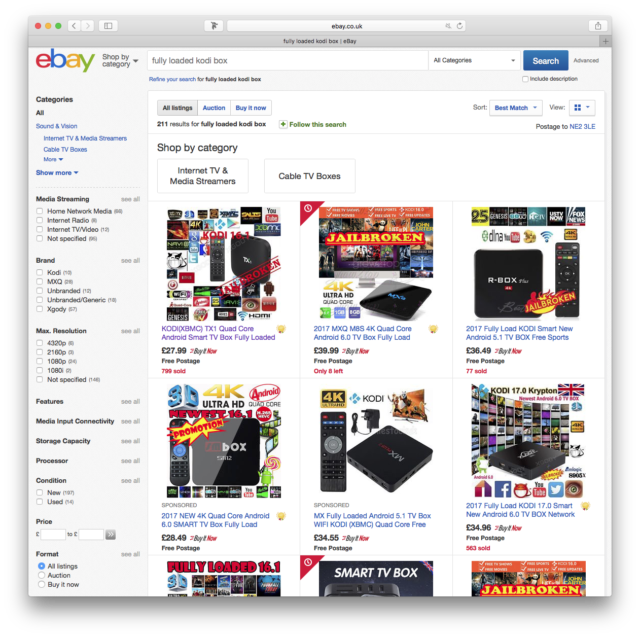This image is a screenshot of an eBay search page. At the very top, there's a gray header featuring three circular buttons in red, yellow, and green, followed by arrows pointing left and right. A search bar at the top displays the URL "eBay.co.uk."

Below the header, against a white background, the interface prominently shows "eBay - Shop by Category." On the left side, categories are listed as follows: All, Sound & Vision, Internet TV & Media Streamers, Cable TV Boxes, with an arrow or pull-down menu beside the word "More." Subcategories include Media Streaming, Home Network Media, Internet Radio, Internet TV & Video, and Non-Specified.

On the right side, prominent buttons offer filtering options such as "All Listings," "Auctions," and "Buy It Now." There's also a sorting option labeled "Sort by Best Match" with a pull-down menu and another control for the view.

In the main content area, the page reveals "211 results for fully loaded Kodi box," with additional navigational cues stating "Shop by Category," "Internet TV & Media Streamers," and "Cable TV Boxes."